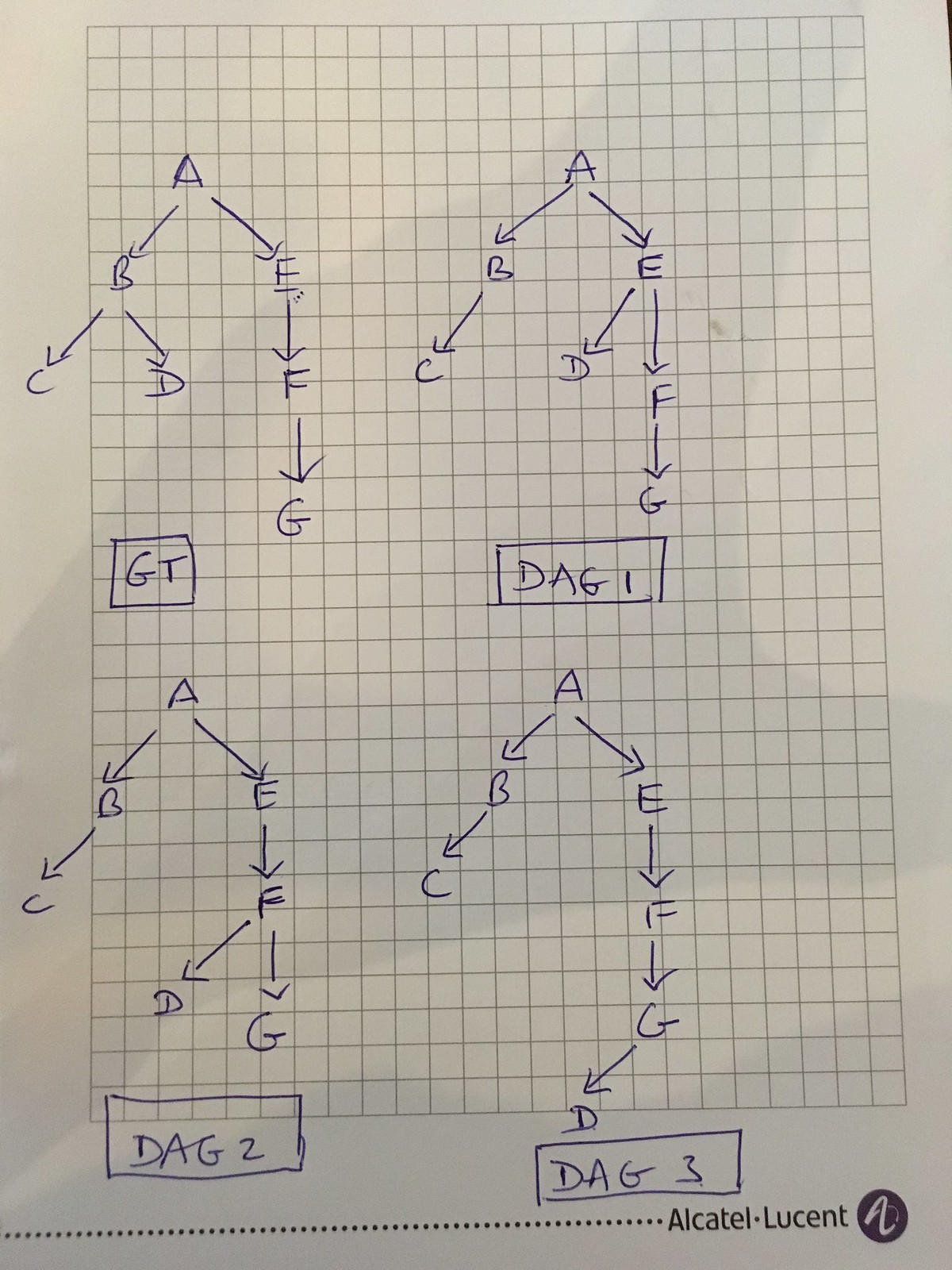This image depicts a piece of graph paper filled with several detailed, interconnected diagrams, all drawn in blue ink. The diagrams resemble complex directed acyclic graphs (DAGs), each labeled and containing various nodes and arrows. 

1. The first graph features connections from:
    - C to B
    - B to D
    - B to A
    - A to E
    - E to F
    - F to G
   This diagram is labeled "GT" at the bottom.

2. The second graph shows pathways from:
    - C to B
    - B to A
    - A to E
    - E to D
    - E to F
    - F to G
   It is labeled "DAG 1".

3. The third graph includes connections from:
    - A to B
    - B to C
    - A to E
    - E to F
    - F to D
    - G
   This graph is labeled "DAG 2".

4. The final graph has routes from:
    - C to B
    - B to A
    - A to E
    - E to F
    - F to G
    - G to D
   This diagram is labeled "DAG 3".

At the bottom of the paper, there is the text "Alcatel Lucent" which might indicate some company affiliation or context.

The entire setup is drawn on graph paper with blue grid lines, conveying a meticulous, handwritten effort to map out these detailed graphs.